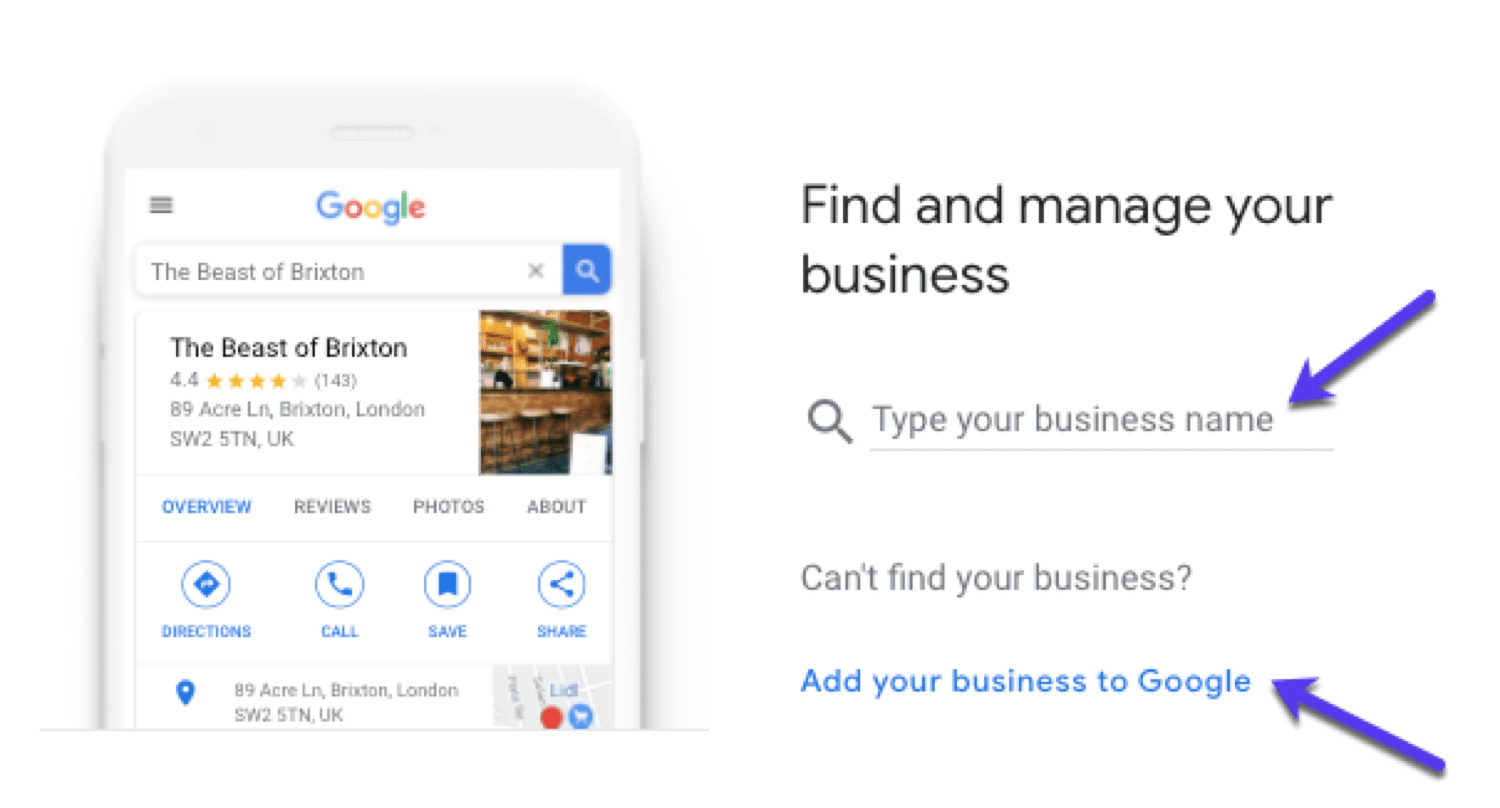The image showcases a person explaining how to use Google to find a business. On the left side, there's a cell phone screen displaying the Google homepage. At the top, the Google search bar contains the typed query "The Beast of Brixton." The search results show "The Beast of Brixton" as a bar/restaurant with a rating of 4.4 out of 5 stars from 143 reviews. A thumbnail image reveals a wooden bar counter with bar stools. The establishment is located at 89 Acre Lane, Brixton, London SW2 5UA, UK. Additionally, the location is marked on a small map.

On the right side of the image, the text "Find and manage your business" is prominently displayed. A purple arrow points to the phrase "Type your business name," indicating where users should input their business information. Below this, there's a question, "Can't find your business?" followed by a blue prompt, "Add your business to Google." Another purple arrow directs attention to this suggestion.